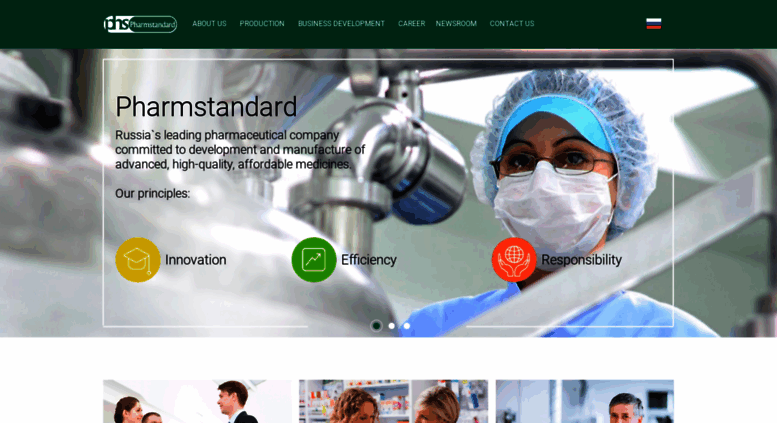Screenshot of a medical website featuring a prominent headline "Farm Standard" positioned slightly to the left. Below the headline, a tagline reads, "Russia's leading pharmaceutical company committed to the development and manufacture of advanced, high-quality, affordable medicines." Directly under this tagline, a section titled "Our Principles" is displayed. This section lists three core values: "Innovation," "Efficiency," and "Responsibility," each accompanied by a corresponding icon that visually represents the respective principle.